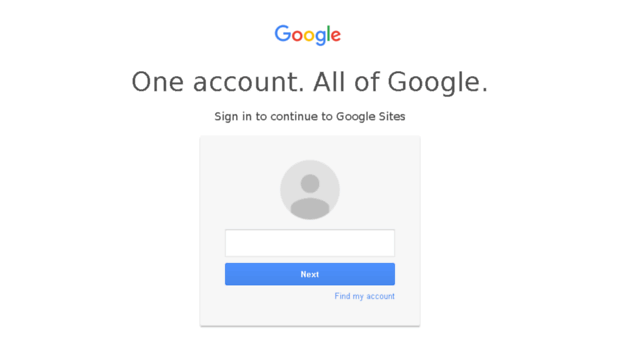The image depicts a Google login screen. At the top, the Google logo is displayed in its signature colors: a blue uppercase "G," a red lowercase "o," a yellow lowercase "o," a blue lowercase "g," a green lowercase "l," and a red lowercase "e." Below the logo, the text reads: "One account. All of Google."

Beneath this, there is smaller text that says, "Sign in to continue to Google Sites." This text is positioned above a light grayish-blue square, approximately four to five inches wide and four inches high. Inside the square, there is a gray circle featuring a darker gray circle within it, representing a placeholder for a user’s profile image.

Underneath these circles, there is an empty rectangle intended for user input. Below this input field, a blue rectangle contains the word “NEXT” in white capital letters. To the right of the blue rectangle, in small blue print, it says "Find my account."